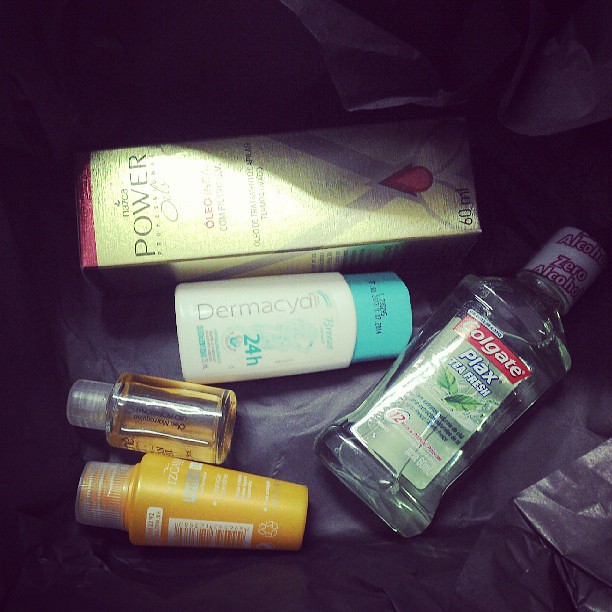The photograph features an array of personal care items meticulously arranged on a black cloth backdrop. At the top left is a long green rectangular box labeled "Power Oleo." Next to it, positioned towards the center, is a white tube with a blue cap labeled "Dermicide." Below the tube sits a small plastic bottle with black writing, containing a light gold liquid. Adjacent to it is another small yellow bottle with a clear cap and white letters. Completing the arrangement on the far right is a clear bottle of Colgate Plax Tea Fresh mouthwash, identifiable by its distinctive branding. The detailed assortment provides a glimpse into a curated selection of beauty and personal hygiene products.